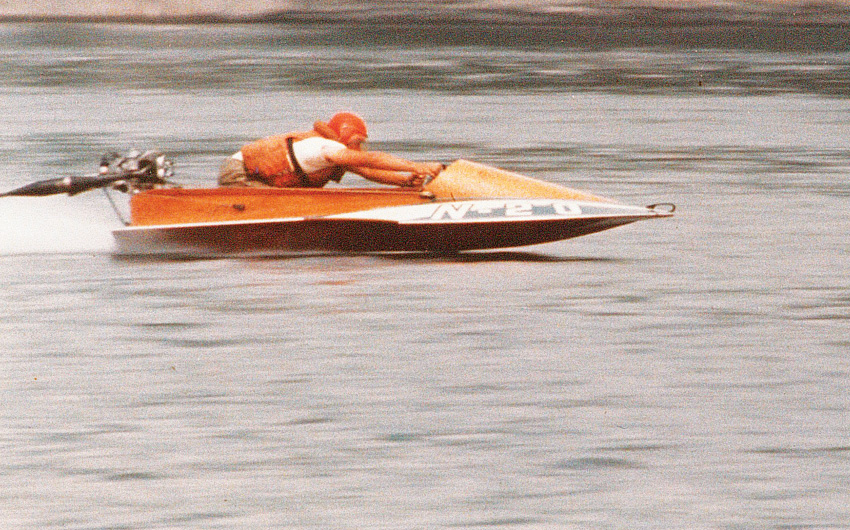This image depicts an action scene on a grayish body of water, possibly a lake or river, where a small orange speedboat, featuring a white stripe on its side panels and the block letters "N20," is zipping through the water. Despite the graininess suggesting it might be an old or low-quality photo, detailed elements are discernible. The boat has a distinctive sharp nose with a black hook or attachment at the front. At the stern, a black motor, also described as silver and thin-pointed in some areas, propels the boat. The rider, clad in an orange helmet that covers the mouth area and an orange life vest over a white t-shirt, with khaki pants or shorts, is fully immersed in the action, gripping the steering wheel with outstretched arms as they navigate the waters. The elevated front of the boat and visible ripples indicate high speed, contributing to an overall dynamic and thrilling atmosphere.